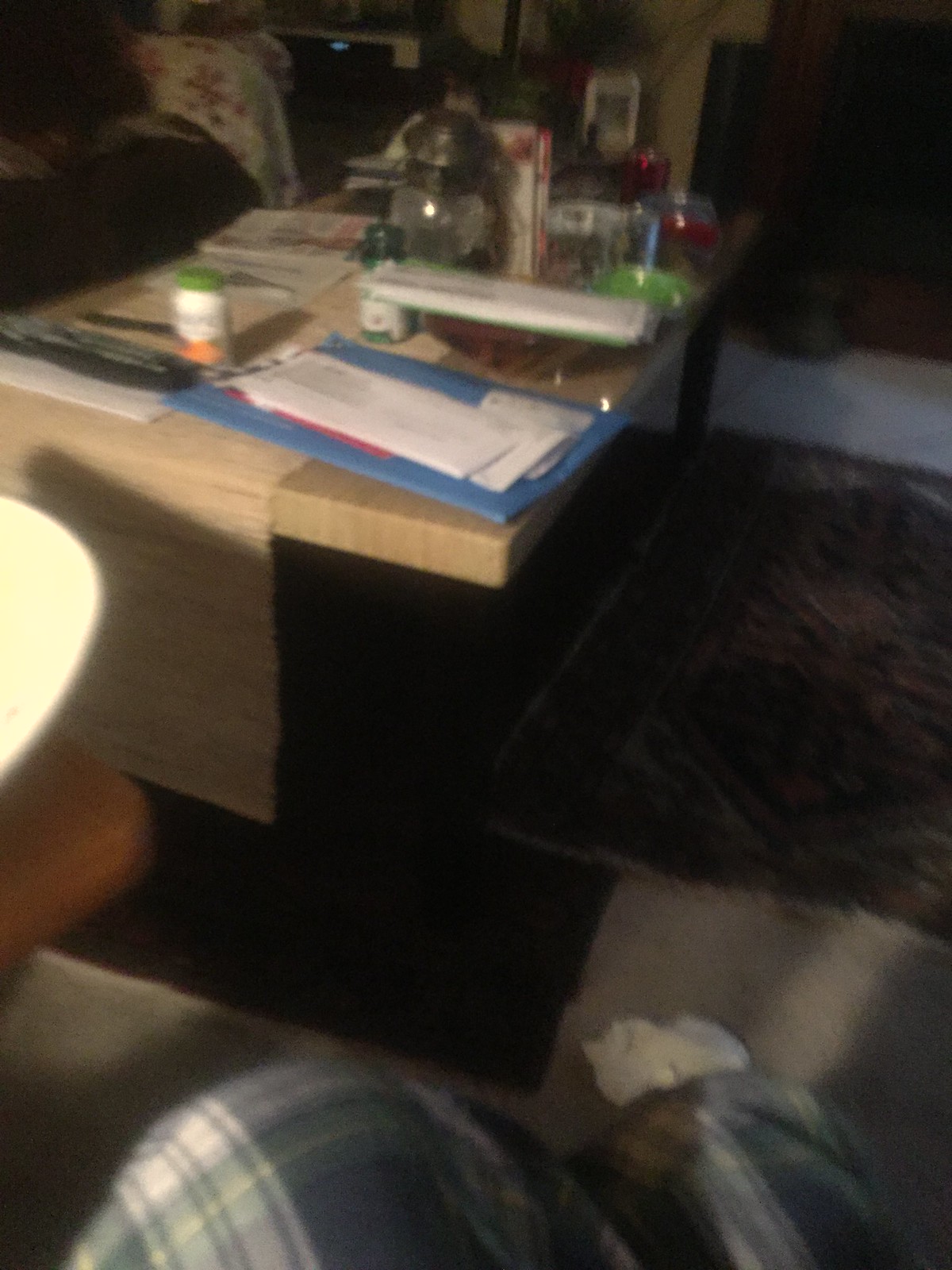This is a somewhat blurry and faded photograph of a cluttered living space. The room features a rug on the floor and a desk that is scattered with various items. The desk holds white envelopes, possibly pieces of mail, a bottle that appears to contain vitamins or medicine, a few books, and some glass bowls. In the foreground, the lower half of a person wearing green and white plaid pajama pants can be seen, with only their knees visible. By their right knee, there is a crumpled tissue. Next to the desk, there is an electronic device that might be a VCR or DVD player. A couch sits nearby, draped with a blanket.